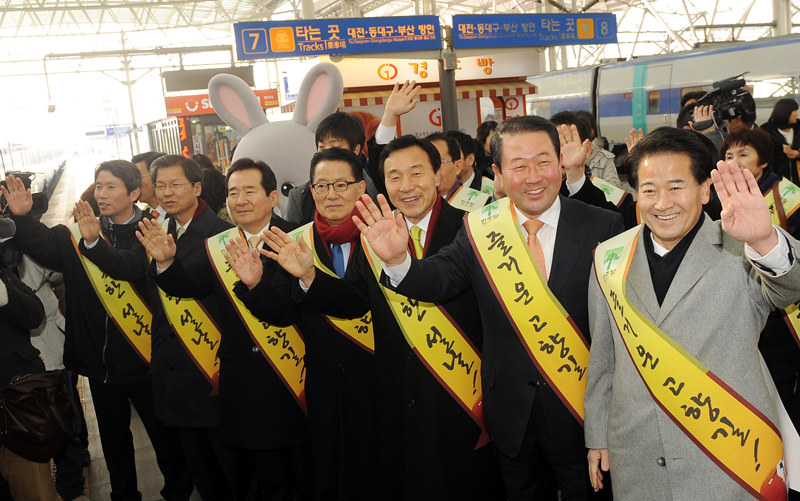The photograph captures a lively scene at what appears to be a train station, likely during an opening ceremony or special event. In the foreground, seven Asian men stand side by side. From left to right, six of them are dressed in black suits with various colored ties, while the man on the far right sports a gray suit. Each man wears a yellow sash adorned with writing that could be either Japanese, Chinese, or Korean. Behind them, a blue and white train can be seen, along with two blue station signs marked with the numbers 7 and 8, and the word "TRAX." To the right, there's a small white building with red markings, possibly a ticket booth. Adding a whimsical touch to the scene, a large bunny mascot and a brown mouse with pink ears are visible in the background, suggesting that they may be part of the festivities. The men appear to be dignitaries, given the formal attire and celebratory mood, with everyone smiling and waving.